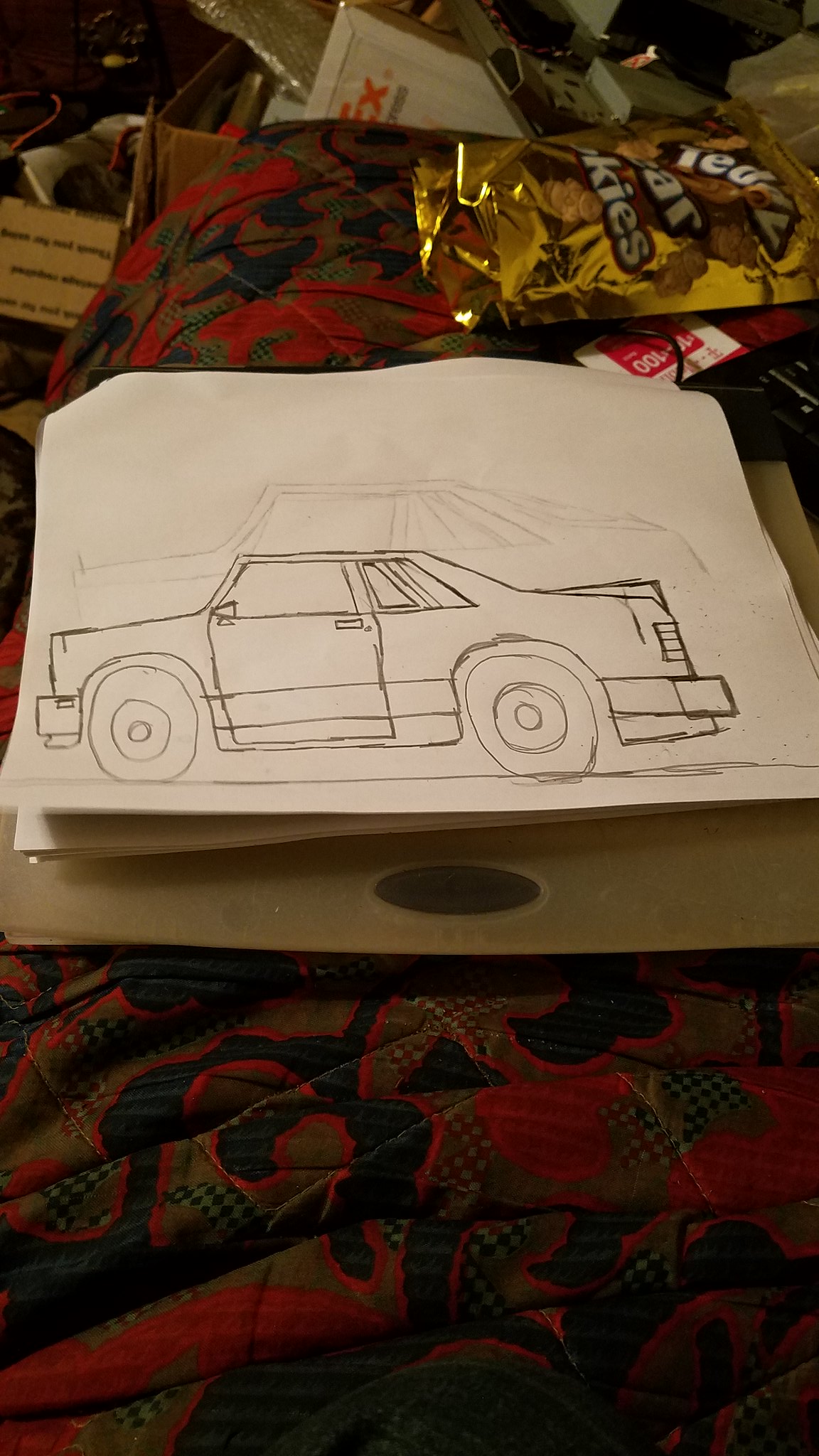This image showcases a detailed, hand-sketched illustration of a mid-sized, two-door car, rendered in black ink or pencil. The car's profile, viewed from the left side, exhibits a boxy design and is placed against a flat brown or gold surface. Intriguingly, a faint, partially erased shadow of a prior drawing of the car is visible just behind and above the current sketch, suggesting it might have been refined multiple times. The car is depicted as driving on a simple line that represents a roadway. The artwork sits atop a comforter or fabric, distinguished by its intricate black, red, yellow, and white patterned design. In the lower part of the image, a gold packet of teddy bear-shaped cookies adds an unexpected, whimsical touch to the scene.